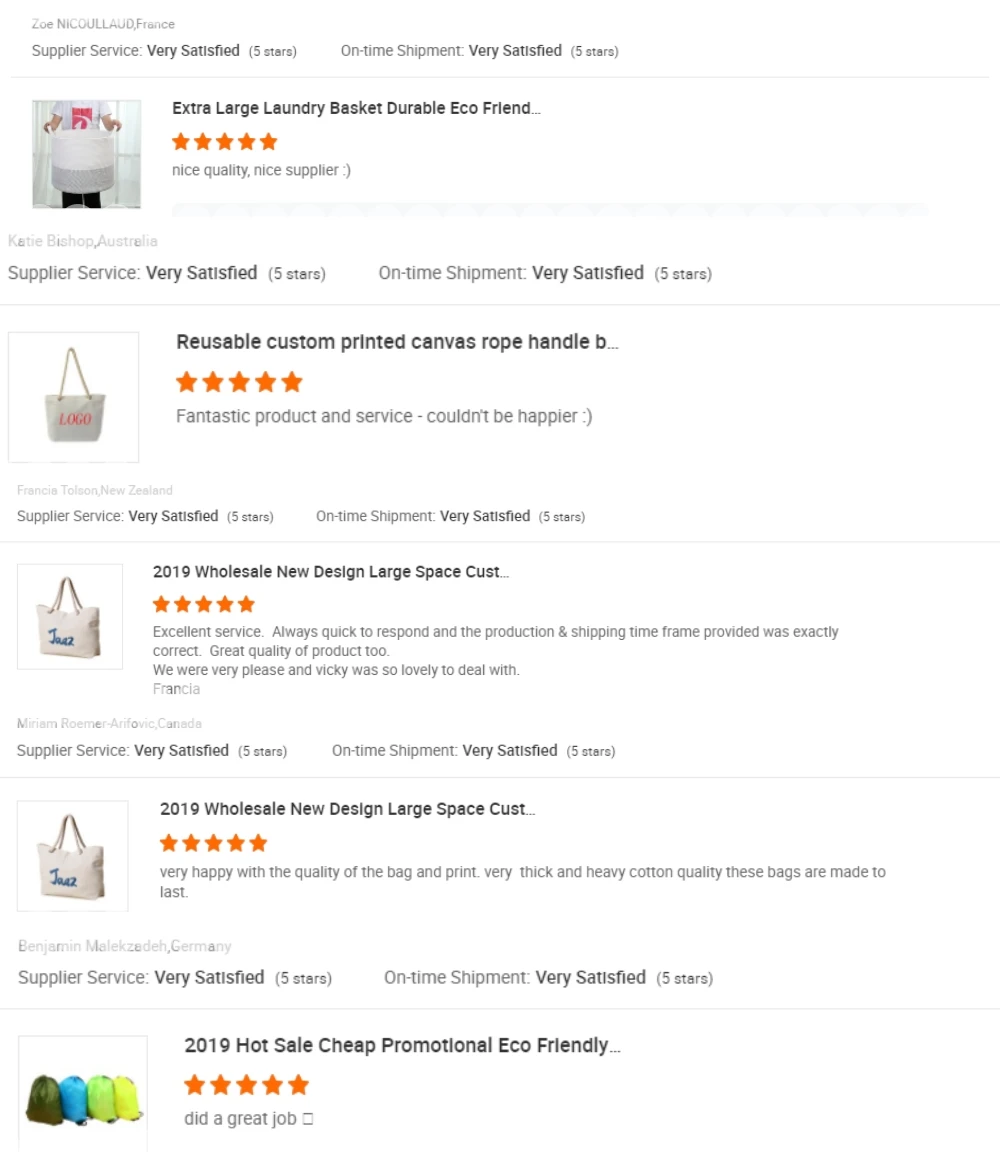The image showcases a screenshot from a website, predominantly featuring user product reviews displayed against a white background with black text. There are several user reviews, each detailing different products along with ratings and comments.

1. **First Review:**
   - **Image:** A man holding a white and gray basket, with his face not visible.
   - **Title:** "Extra Large Laundry Basket, Durable, Eco-Friendly"
   - **Rating:** ★★★★★ (5 stars)
   - **Description:** "Nice quality, nice supplier."
   - **Supplier Service Rating:** Very satisfied
   - **On-Time Shipment Satisfaction:** Very satisfied

2. **Second Review:**
   - **Image:** A white tote bag
   - **Title:** "Reusable Custom Printed Canvas Rope Handle..."
   - **Rating:** ★★★★★ (5 stars)
   - **Description:** "Fantastic product and service, couldn't be happier."
   - **Supplier Service Rating:** Very satisfied
   - **On-Time Shipment Satisfaction:** Very satisfied

3. **Third Review:**
   - **Image:** A white tote bag positioned slightly off-center
   - **Title:** "2019 Wholesale New Design, Large Space, Cust..."
   - **Rating:** ★★★★★ (5 stars)
   - **Description:** "Excellent service, always quick to respond, and the production and shipping time frame provided was exactly correct. Great quality of product too, we were very pleased, and Vicky was so lovely to deal with."
   - **Supplier Service Rating:** Very satisfied
   - **On-Time Shipment Satisfaction:** Very satisfied

4. **Fourth Review:**
   - **Image:** The same off-center white tote bag
   - **Title:** "2019 Wholesale New Design, Large Space, Cust..."
   - **Rating:** ★★★★★ (5 stars)
   - **Description:** "Very happy with the quality of the bag, in print, very thick and heavy cotton quality, these bags are made to last."
   - **Supplier Service Rating:** Very satisfied
   - **On-Time Shipment Satisfaction:** Very satisfied

5. **Fifth Review:**
   - **Image:** Four different green and blue colored bags
   - **Title:** "2019 Hot Sale Cheap Promotional Eco-Friendly..."
   - **Rating:** ★★★★★ (5 stars)
   - **Description:** "Did a great job."
   - **Supplier Service Rating:** Not specified
   - **On-Time Shipment Satisfaction:** Not specified

This detailed breakdown provides a clear and comprehensive overview of the product reviews, highlighting the users' satisfaction with both the products and the supplier services.